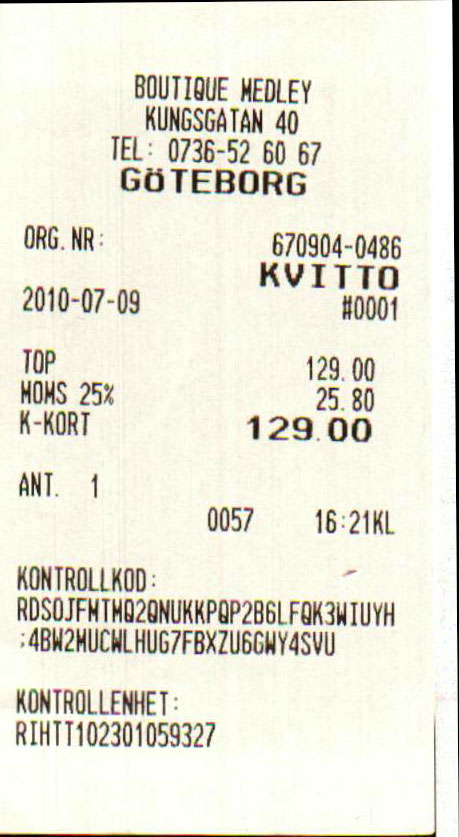This image shows a detailed receipt likely from a shop or possibly a petrol station in Gothenburg, Sweden. The entire document is in Swedish, making it somewhat challenging to decipher without linguistic knowledge. The receipt totals 129 Swedish Krona (SEK), indicating it reflects purchases made on site. The transaction date is either July 7, 2010, or September 7, 2010, depending on the date format used. The rest of the receipt contains numerous unreadable lines of Swedish text, likely detailing items purchased and other transaction specifics.